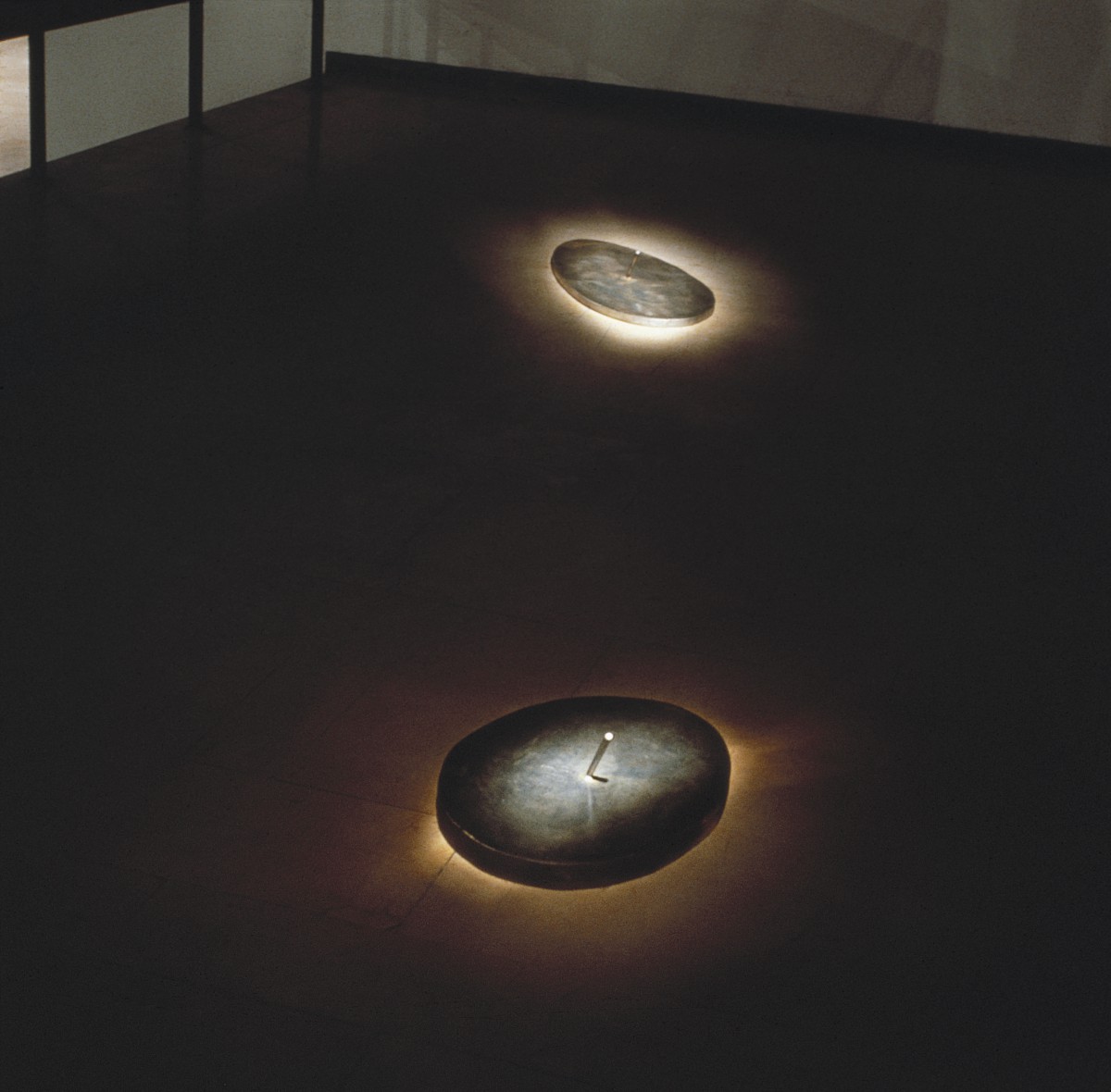The painting depicts a dimly lit, modern room with a dark brownish floor that lightens towards the forefront and darkens towards the back. The focal point of the scene features two oval-shaped disks, one positioned towards the upper middle and the other towards the lower middle of the composition. These disks appear to be black with central sticks and a white dot at the tip, which might be pins holding them to the floor. Beneath each disk, a radiant, almost glowing white light is trying to escape, casting a mystical illumination in the otherwise dark room. The background reveals white paneled walls accented with brown or black columns, adding a structural element to the space. The overall painting has a realistic quality that momentarily makes one question if it might be a photograph. The detailed portrayal and play of light suggest an intriguing modern piece that is nearly square in shape.